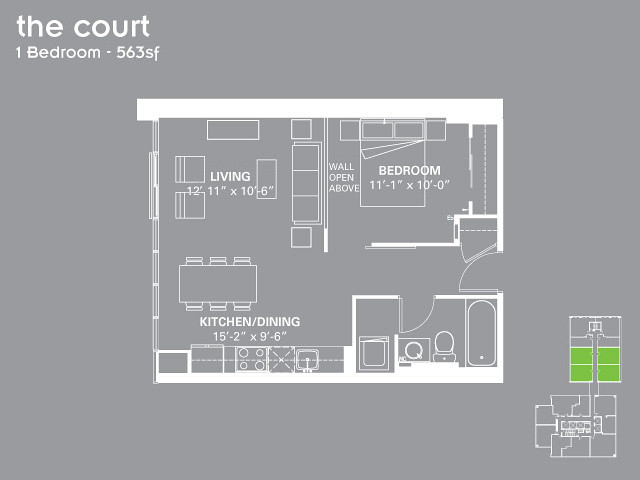The image is a detailed floor plan for a condominium unit named "The Court," which features one bedroom and occupies 563 square feet. The diagram is elegantly rendered in white against a dark gray background, utilizing a clean sans serif font throughout for a modern, easy-to-read presentation.

The layout highlights several distinct areas within the unit, including a living room, bedroom, kitchen/dining room, and bathroom. The living room measures 12 feet 11 inches by 10 feet 6 inches, furnished with symbols representing a couch, two armchairs, two end tables, a coffee table, and a sideboard. Adjacent to the living room, the bedroom is slightly smaller at 11 feet 1 inch by 10 feet, featuring a bed with two pillows, two night tables, and two closets—one spanning the full length of a wall and the other being a smaller, walk-in closet.

The kitchen/dining area measures 15 feet 2 inches by 9 feet 6 inches and includes depictions of a stove, sink, and refrigerator. Additionally, there is a graphic indicating a dining table with seating for six people. Centrally located, and visible from both the bedroom and the hallway leading to the kitchen/dining area and the exterior entrance, is the bathroom. This space is equipped with a tub, vanity, and toilet.

Adjacent to the bathroom, there is a smaller, unnamed area that could potentially serve as a linen closet or house a laundry unit, though its specific function is not detailed. The bottom right portion of the image includes drawings of what appears to be a larger section of the condominium complex. This section contains four bright green panels; however, their exact purpose remains unspecified.

Overall, this floor plan offers a comprehensive visualization of "The Court," illustrating both the unit's spatial organization and its potential furnishing layout.